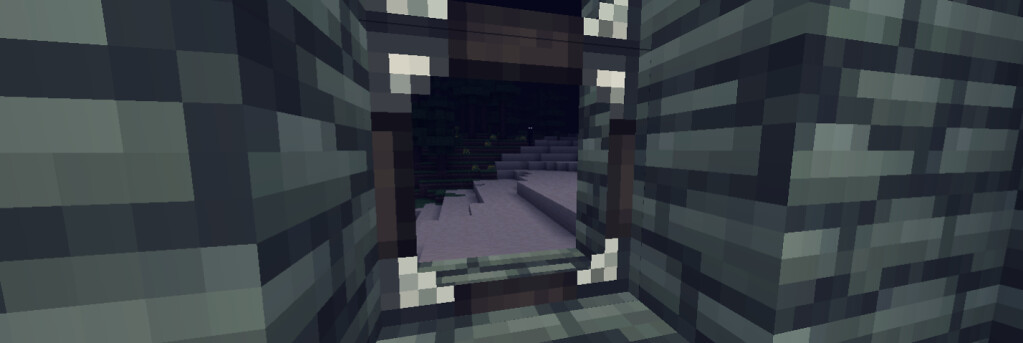The image appears to be a screenshot from a video game, likely Minecraft, characterized by its pixelated graphics. It presents a close-up view of two distinct sections or rooms. The initial room features walls made of stone blocks that exhibit a patterned mix of light gray, dark gray, greenish-gray, and black colors. On the left and right sides of this room, there are additional walls in similar shades. The focal point of the image is an inset window or doorway located centrally, framed by gray, brown, and white hues. Beyond this opening, the scene reveals purplish steps or stairs amidst more block walls. The background visible through the window suggests a night sky, depicted with varying shades of purple and black. The entire scene is detailed with the game's characteristic low-resolution, pixelated texture, adding to the stylized, yet somewhat unclear nature of the visuals.